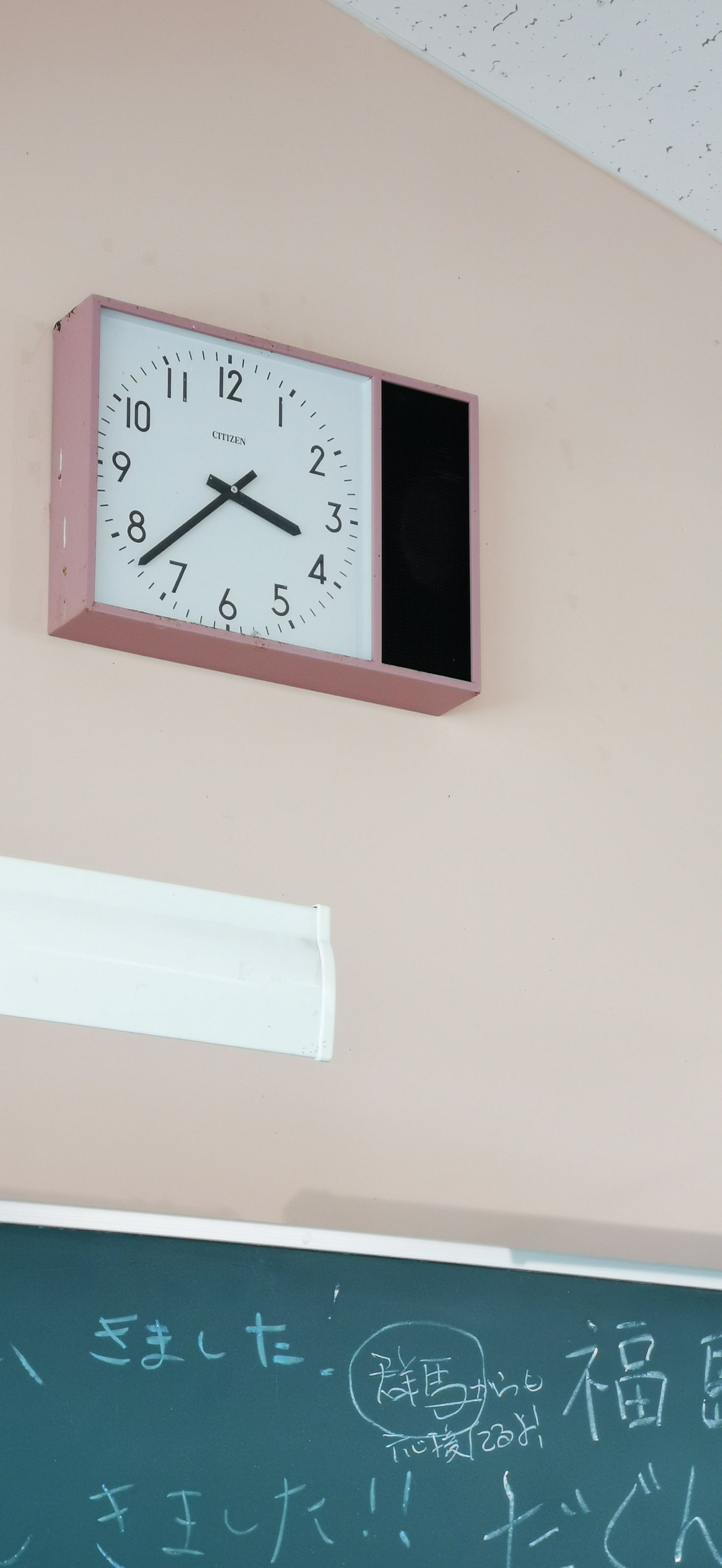In this classroom scene, the walls are painted a soft pink hue, contrasting with the crisp white ceiling overhead. Prominently featured on the pink wall is a distinctive white line, possibly marking an air vent or some kind of wall fixture. A pink clock adorns the wall as well, its design incorporating a white face with clear, black numerals and black hands, set against a small black section on the right side. Below this clock, a green chalkboard with silver trim can be seen, covered in various handwritten equations and words in white chalk.